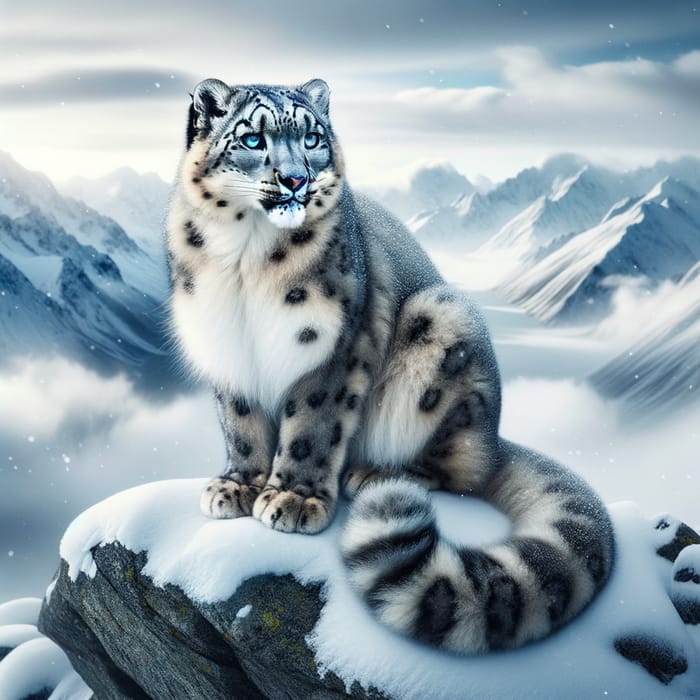In this artist's rendition, a majestic snow leopard is depicted sitting regally on a snow-covered rock, surrounded by vast mounds of snow and an expansive, cloud-filled sky with a hint of blue and occasional stars. The leopard, characterized by its striking light blue eyes and predominantly gray fur, features a white underbelly adorned with black spots. Its nose, primarily black with a hint of pink, and the black stripes around its eyes and on the top of its head, add to its distinguished appearance. The animal's large, fluffy tail, marked by broad black stripes, curls gracefully around its body. The leopard's neck and chest showcase a white 'bib' with black speckles, extending up towards its more grayish face. The serene backdrop, possibly inspired by the snowy peaks of a place like Mount Everest, combines with the foggy valley below and thick clouds above, creating a striking yet tranquil scene where the snow leopard dominates the image with its alluring, almost ethereal presence.